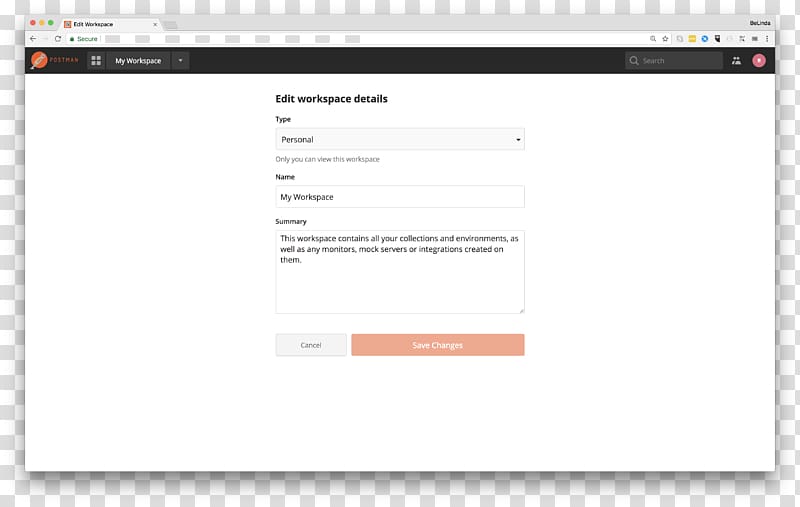A Mac computer displays a website on its screen, identifiable by the characteristic macOS window control buttons in the upper left corner: a red button for closing, a yellow button for minimizing, and a green button for maximizing the window. Only one tab is open, but the tab label is unclear. Below the tab bar, familiar navigation controls are visible: a left-facing back arrow, a refresh button, and a small, hard-to-read text that seems to indicate the page is secure.

The interface below features a black banner stretching across the screen. On the left side of the banner, an orange logo is visible next to a drop-down menu labeled "My Workspace." To the far right, there is a search field and a user icon inside a pinkish-red circle.

Further down, against a white background, the user interface displays the title "Edit Workspace Details" in black font. Below this title, labeled fields and input areas include "Type" with a drop-down menu currently set to "Personnel," and "Name" with a text field displaying "My Workplace." The "Summary" section contains some text, details of which are unspecified. At the bottom of this section, two buttons are positioned side-by-side: an orange "Save Changes" button and a "Cancel" button.